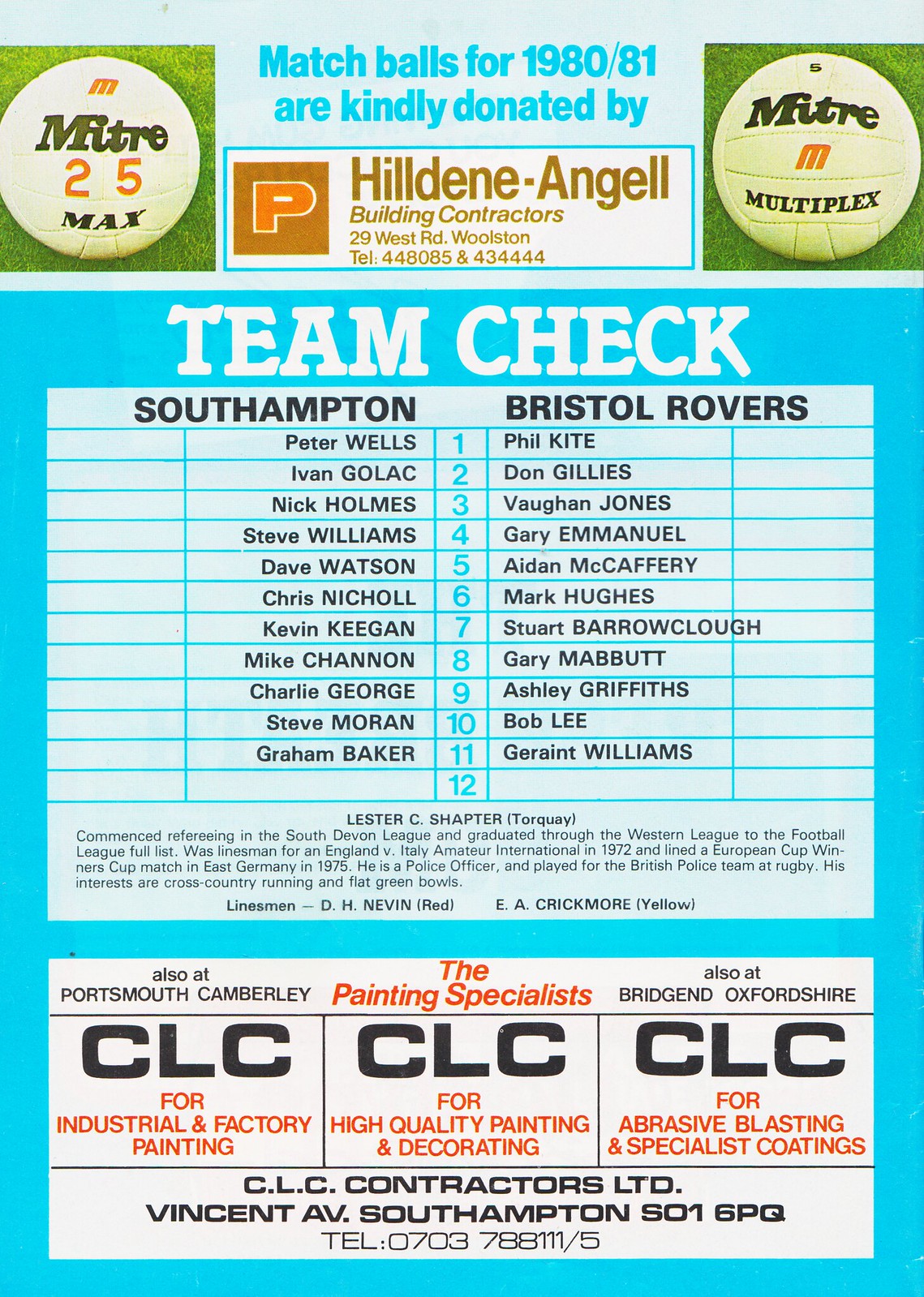This image is a scanned page from an early 1980s football (soccer) program, primarily dominated by light blue hues. At the top, there is an advertisement for Hildene-Angel, building contractors located at 29 West Road, Wollaston, with their phone number provided. They are acknowledged for donating match balls for the 1980-81 season. Flanking this ad are two inset photographs of footballs on grass; both feature the Mitre logo and branding, with one labeled "Mitre 25 Max" and the other "Mitre Multiplex."

The central section, marked by a prominent "Team Check" heading in large white letters against a light blue background, lists the player lineups for Southampton and Bristol Rovers. Southampton's roster, numbered 1 through 11, includes Peter Wells, Ivan Golac, Nick Holmes, Steve Williams, Dave Watson, Chris Nicholl, Kevin Keegan, Mike Channon, Charlie George, Steve Moran, and Graham Baker, with the 12th slot left blank. Bristol Rovers' lineup features Phil Kite, Don Gillies, Vaughan Jones, Gary Emanuel, Aiden McCaffery, Mark Hughes, Stuart Barrowclough, Gary Mabbutt, Ashley Griffiths, Bob Lee, and Geraint Williams, similarly leaving the 12th position unfilled.

Beneath the team lists, in small print, are player particulars and a blue border. At the bottom of the page, another advertisement appears for CLC Contractors Limited, specializing in industrial and factory painting, high-quality painting and decorating, and abrasive blasting and specialist coatings. CLC has offices in Southampton, Portsmouth, Camberley, and Bridgend, Oxfordshire, with their contact details included. This entire page, framed in a sky blue background, is a snapshot of a football match program from the early 1980s.